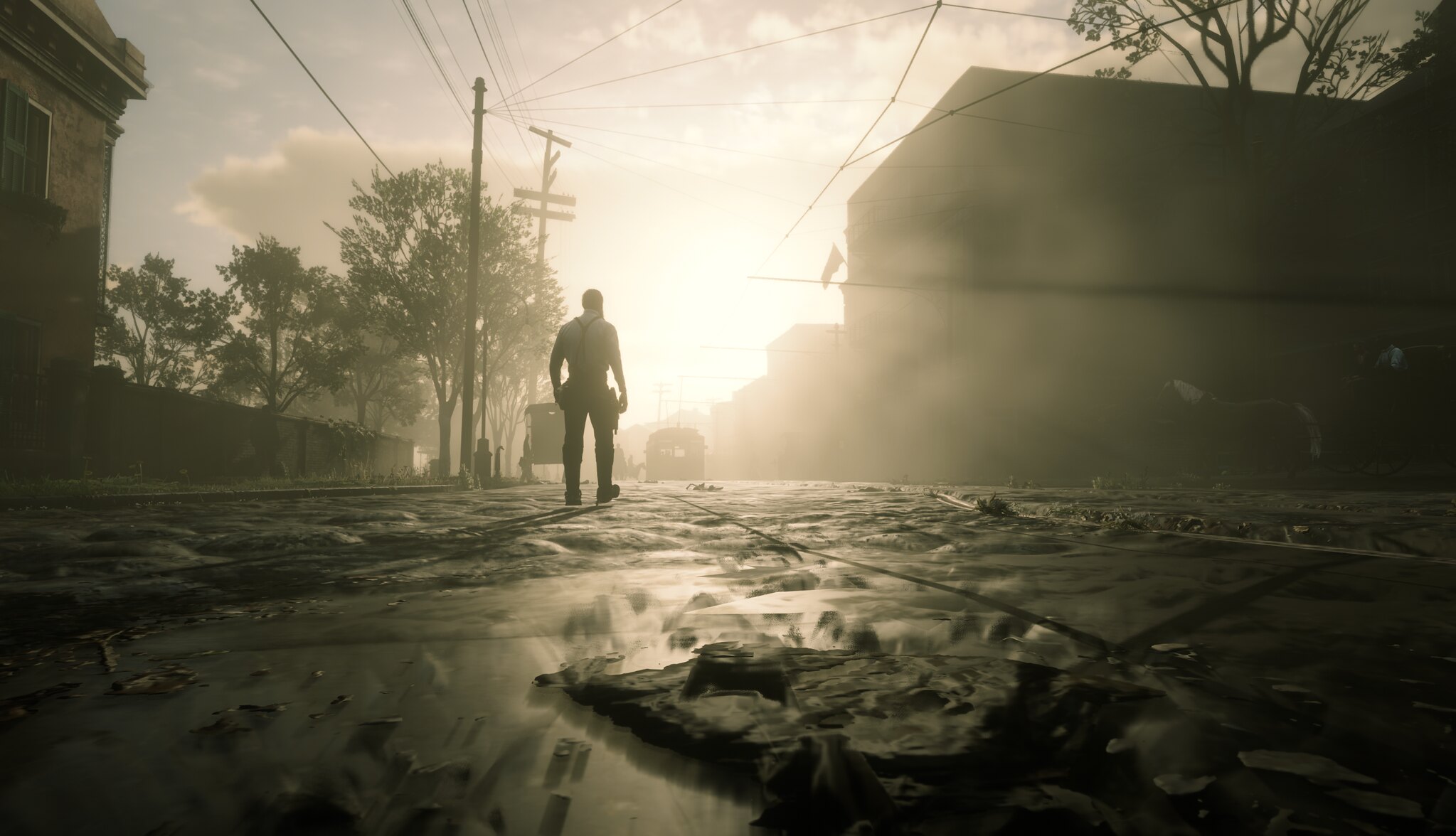The image captures a hazy morning or evening scene, possibly during sunrise, set in the world of Red Dead Redemption. The atmosphere is thick with fog, creating an ethereal glow as the light breaks through the horizon, casting long shadows and illuminating the sky with subtle pastel hues. In the foreground, the ground, whether covered in snow or littered debris, adds to the rough texture of the scene. Centered in the frame and just slightly to the left, a solitary figure walks down a litter-strewn road, his silhouette accentuated by the hazy backdrop. The man, dressed in blue jeans and suspenders, is viewed from behind, adding a sense of mystery and solitude. On either side of the road, buildings line up with visible facades—brick on the left and several structures on the right—while deciduous trees stretch their branches into the misty air. Power lines and poles run parallel along the road, connecting the scene to the rustic aesthetic of the game. In the distance, a faint silhouette of a flag can be seen fluttering, and a vehicle appears further down the road, hinting at the settled yet lively nature of the town.